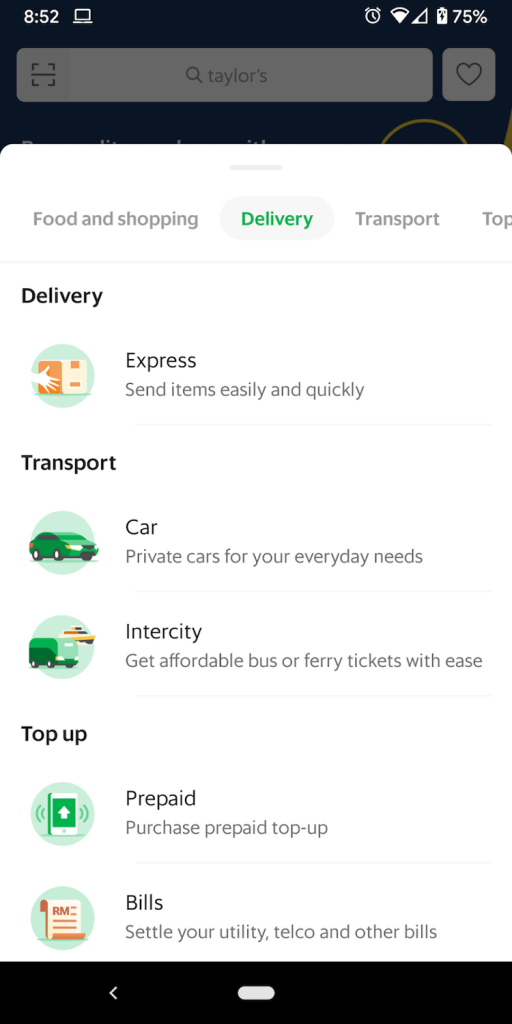**Category: Websites**

**Caption:**

The phone screen displays the time as 8:52 and indicates that an alarm is set. The signal bars are low, but Wi-Fi is being utilized, and the battery level is at 75%. Just below the status indicators, there is a search bar with the word "tailors" entered. Adjacent to the search bar, there is a heart icon for favoriting options.

Beneath the search bar, there are categorized options including "Food and Shopping" in gray, "Delivery" in green, "Transport" in gray, and "Top" in gray. Below these categories, a line separates the main content section. 

Under the "Delivery" section, an icon depicts a white hand holding an orange and white box against a blue circular background. The section details various services:
- **Express:** Send items easily and quickly.
- **Transport:** Car, private cars for your everyday needs.
- **Inner City:** Get affordable bus or ferry tickets with ease.
- **Top Up:** Prepaid, purchase prepaid top-ups.
- **Bills:** Settle your utility, telco, and other bills.

This interface provides a comprehensive menu for various services, suitable for daily tasks and errands.